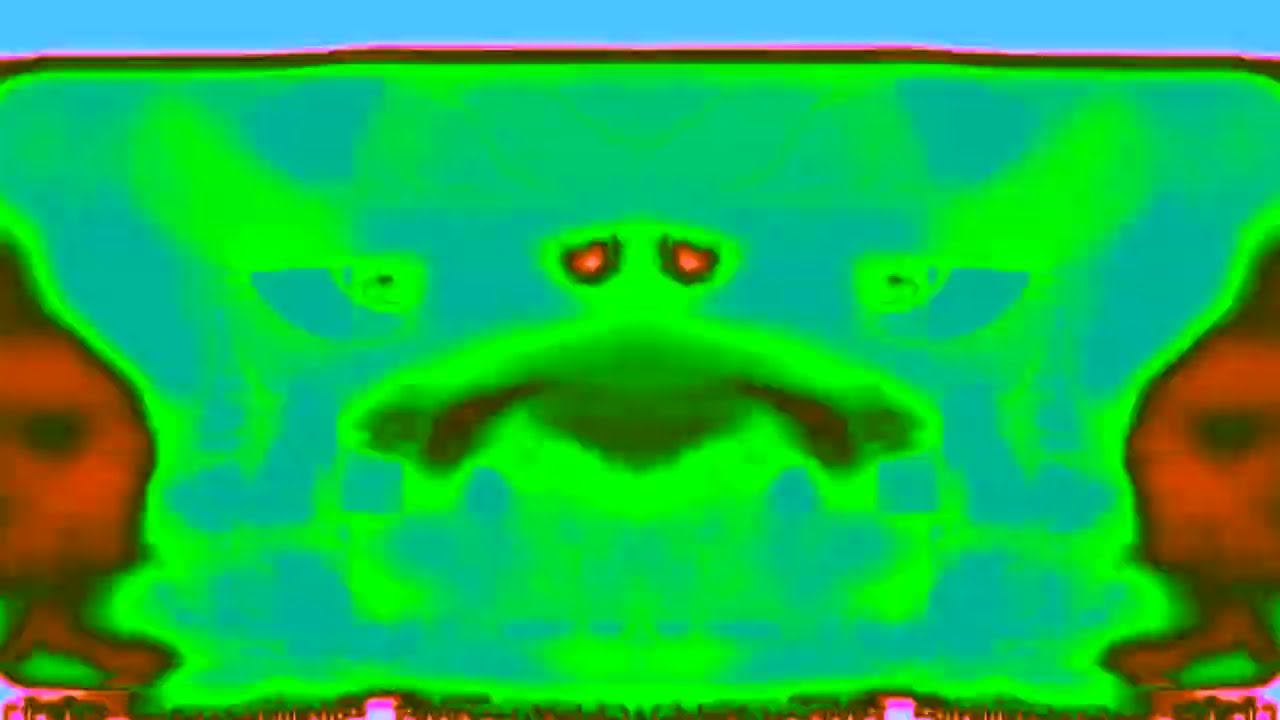The image features a green, blob-like creature with red, heart-shaped eyes positioned centrally against a dynamic, vortex-like green background. The creature, resembling a frog, exudes a digital, low-graphic quality typical of video game screenshots. Flanking this central figure are two red characters, seemingly more abstract with large pointed heads and legs, without distinct bodies, giving them a delicate appearance. Both characters have black eyes and contribute to the image's shadowy aesthetic. The scene is bordered by pink hues at the top and bottom, accompanied by blue accents, enhancing the overall digital and slightly blurry appearance. The pink border emerges prominently at the top, contrasting with an aqua-colored central area that suggests the creature's darker middle or limbs. Some cut-off words are visible below the figures, reinforcing the screenshot-like quality of this illustration.